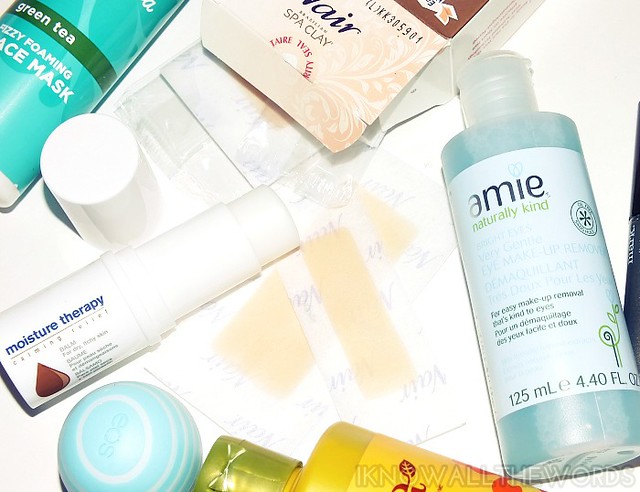The color photograph showcases a variety of cosmetic products arranged on a clean, white background. On the left side of the image, there is a plastic bottle filled with an aqua-colored liquid. It features a white label that reads "Ami, naturally kind" and specifies its use for easy makeup removal with the phrase "that's kind eyes," written in both English and another language. 

To the right of this bottle, tan-colored wax removal strips are neatly placed. Above these strips, the upper portion of a box of Nair spa clay is visible, though most of it is cropped out of the frame. Further right, a partially cropped tube of green tea fizzy foaming face mask is seen. The tube is aqua with an olive green stripe across it.

Additionally, there is a moisture therapy calming relief balm lying on its side, with its white cap detached and resting next to it. At the very bottom of the image, a yellow bottle with red design details is visible but heavily cropped, making it difficult to discern specific details.

Finally, a distinctive blue sphere embellished with white concentric circles, which appears to be a lip balm, completes the arrangement of products in the photograph.